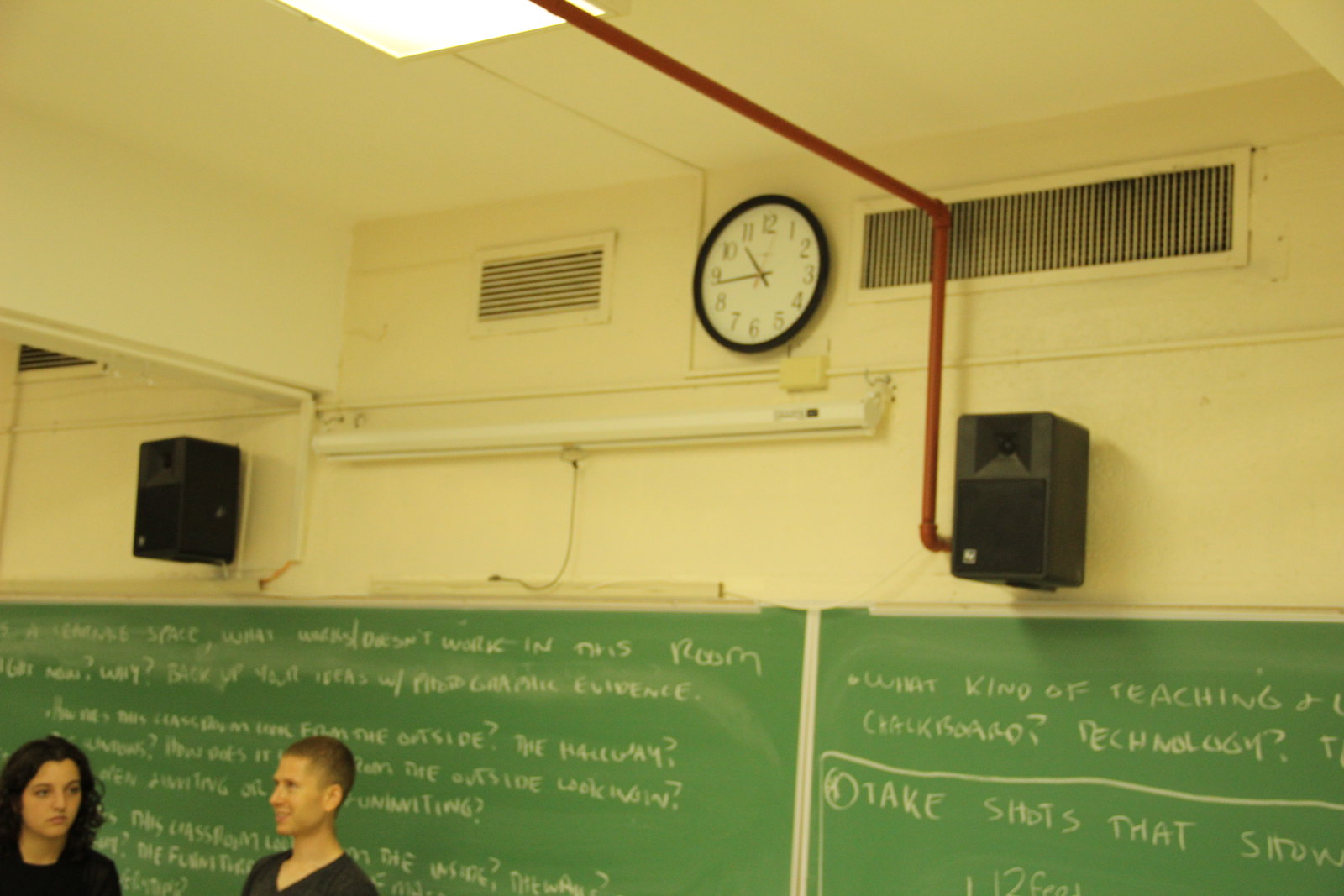The image is a color photograph of a classroom interior, taken with an older camera or phone, evident from its slightly blurry quality and coloring. The yellowish walls feature a clock with a black plastic casing and a white face, showing the time as approximately 10:44. Above the green chalkboard, which stretches across the bottom of the image, there are vents and speakers, along with a closed pull-down projection screen. The chalkboard is filled with various writings, mostly illegible. In the bottom left corner, two people are standing in front of the chalkboard. On the left is a young woman with long black hair, facing forward without any expression, and to the right is a young man with a buzz cut and a black v-neck t-shirt, smiling and facing towards the left. The scene suggests they might be presenting something.